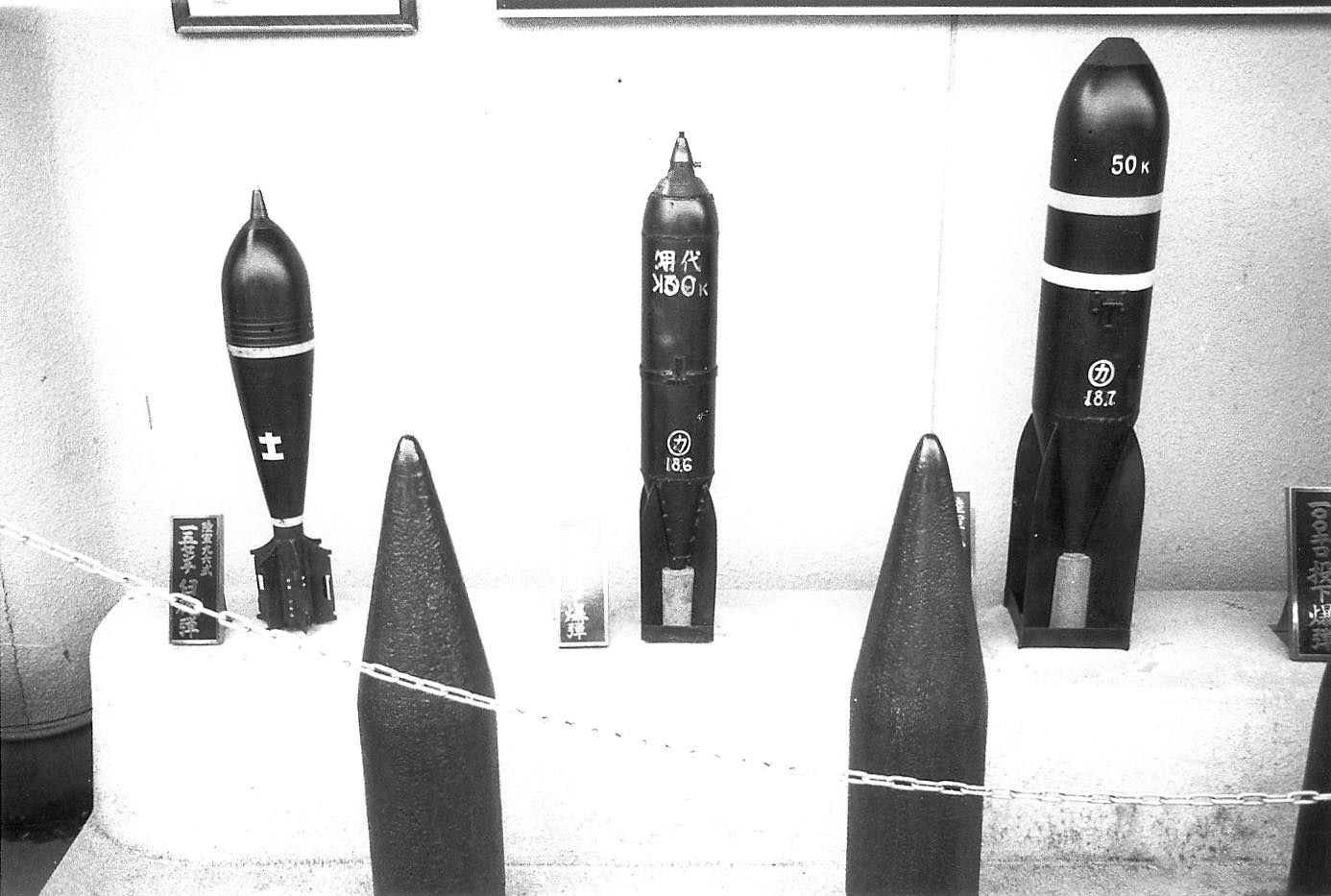This detailed black-and-white photo showcases an exhibit likely situated in a war museum. The scene features various bombs and artillery shells displayed prominently on a white, possibly concrete, platform. The display is bordered by a chain or metal rope, ensuring visitors maintain a respectful distance.

In the front row, there are three distinct artillery shells, resembling massive, elongated bullets, each several feet tall. These are each accompanied by descriptive plaques written in what appears to be Asian, likely Chinese, characters. Behind them, on the elevated platform, are additional bombs that appear to be deactivated.

From left to right, the exhibit starts with the smallest bomb, which is black and has a more rounded top tapering downwards. The middle bomb is of a consistent cylindrical shape and slightly taller. The tallest bomb on the right stands out with white stripes and bears the marking "50k," hinting at a significant measurement, possibly 50 kilograms or 50 kilotons.

The background includes a white, concrete-like wall with framed images visible at the bottom, lending a stark and historical atmosphere to the setting. The meticulous layout and Asian inscriptions imply the relics could be from historical conflicts, emphasizing the solemn significance of the exhibit.